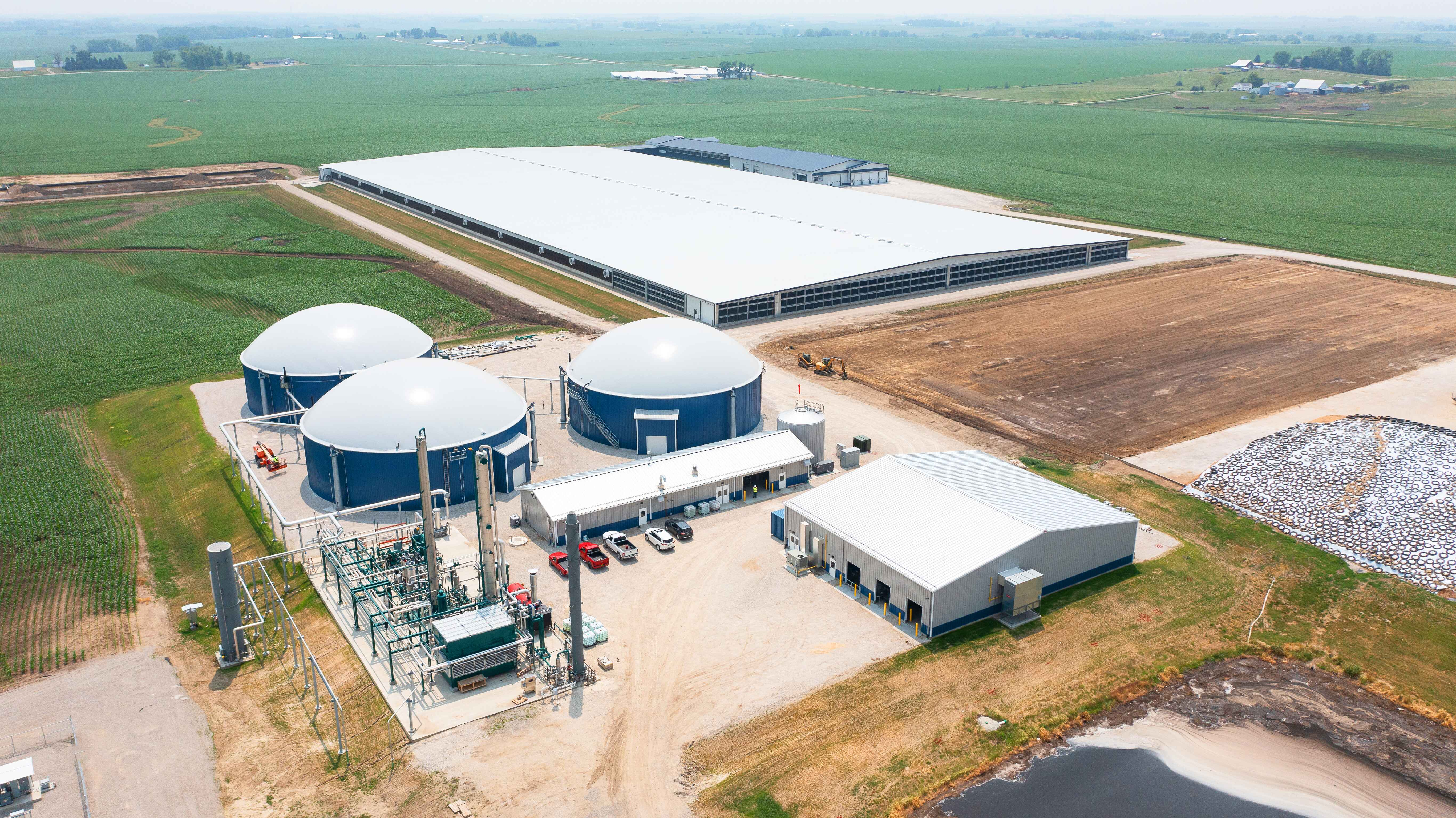This detailed aerial image, likely taken from a drone or high vantage point, reveals an extensive industrial facility set amidst expansive green fields and cleared lands. The central feature is a large, one-story building with a white roof, possibly a factory or farm structure. Adjacent to this, there is a brown field and a trio of circular blue structures with white roofs, which might be silos, oil drums, or research stations.

In the foreground, a long rectangular building fronts a parking area filled with trucks, while nearby, a medium-sized square building with an attached air conditioning unit is noticeable. To the right, an intricate arrangement of large metal pipes, possibly for electrical or fluid transport, is enclosed by a fence or gate. The bottom-right corner also hints at some water or runoff associated with the facility. The image, captured in foggy daylight conditions, lacks visible signage identifying the company or specific purpose of the structures.